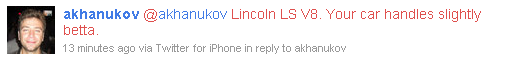The image is a screenshot of a Twitter reply displayed on a predominantly white background. On the left side of the image, there is a small square avatar of a smiling Caucasian man with short brown hair, slightly cropped, and a hint of facial hair. The avatar has a black background, making the man’s face the focal point. To the right of the avatar, the text appears with the handle "A-K-H-A-N-U-K-O-V" written in blue, followed by the same handle prefixed by an @ symbol also in blue. The reply reads in red, "a lincoln lsv8 your car handle slightly betta," with "betta" spelled as B-E-T-T-A. Below this message, in smaller black text, it states "13 minutes ago via Twitter for iPhone in reply to A-K-H-A-N-U-K-O-V." This neatly structured Twitter reply captures the concise interaction on the social media platform.